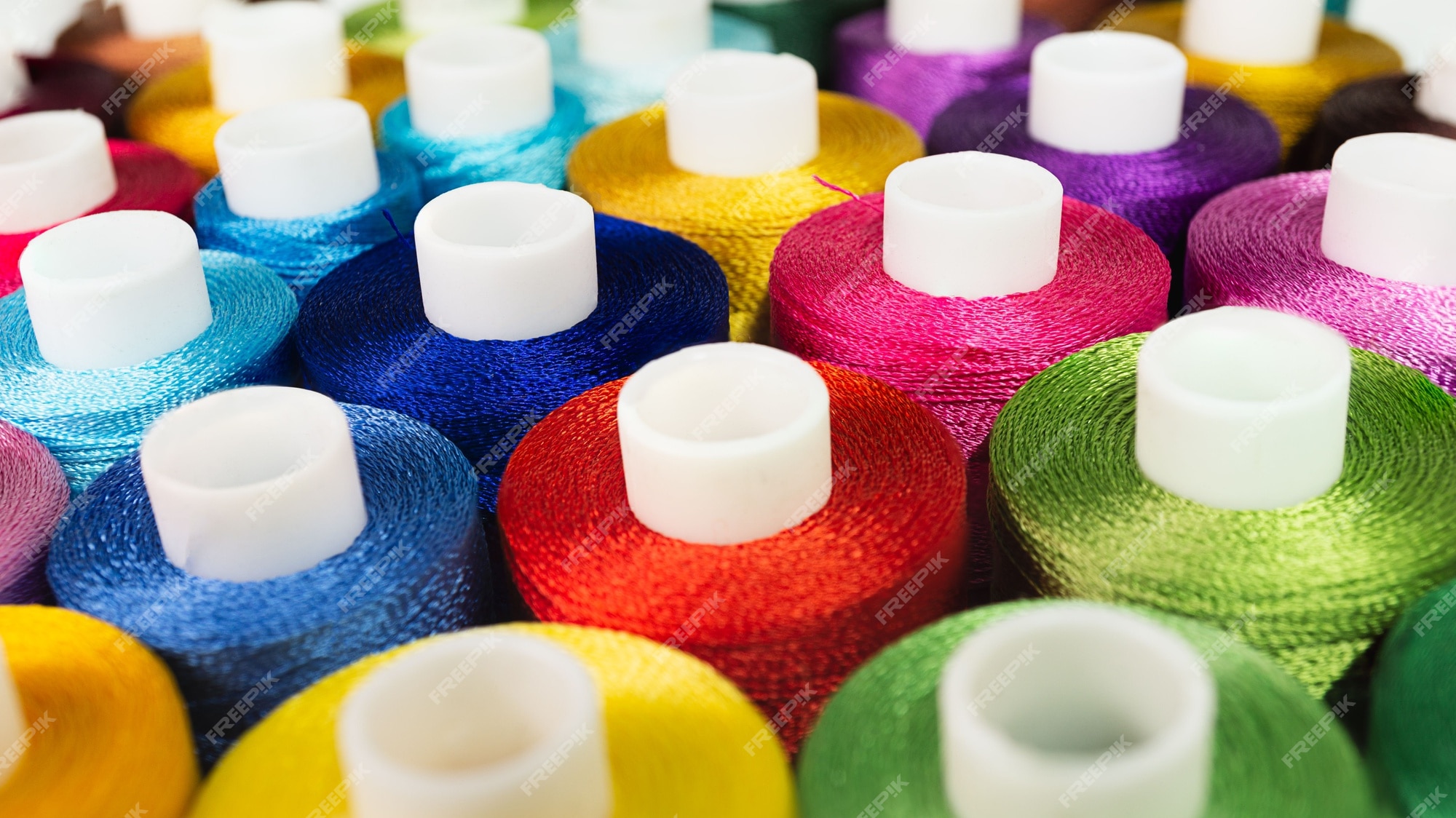A close-up view captures a vibrant array of spools of thread, neatly positioned close to each other. The spools feature a variety of colors, including different shades of blue ranging from cyan to navy, as well as red, pink, light green, dark green, yellow, magenta, gold, and purple. Each thread is meticulously wound around a white plastic cylinder. The image employs a shallow depth of field, focusing sharply on a few central threads while the foreground and background blur gently. This enhances the texture and vividness of the spools, making them appear almost tactile. Adding to the composition, there is a semi-transparent diagonal watermark with the text "free pick." Overall, it seems like these spools, possibly used for machinery or crafting, offer a rich display of colors and textures.